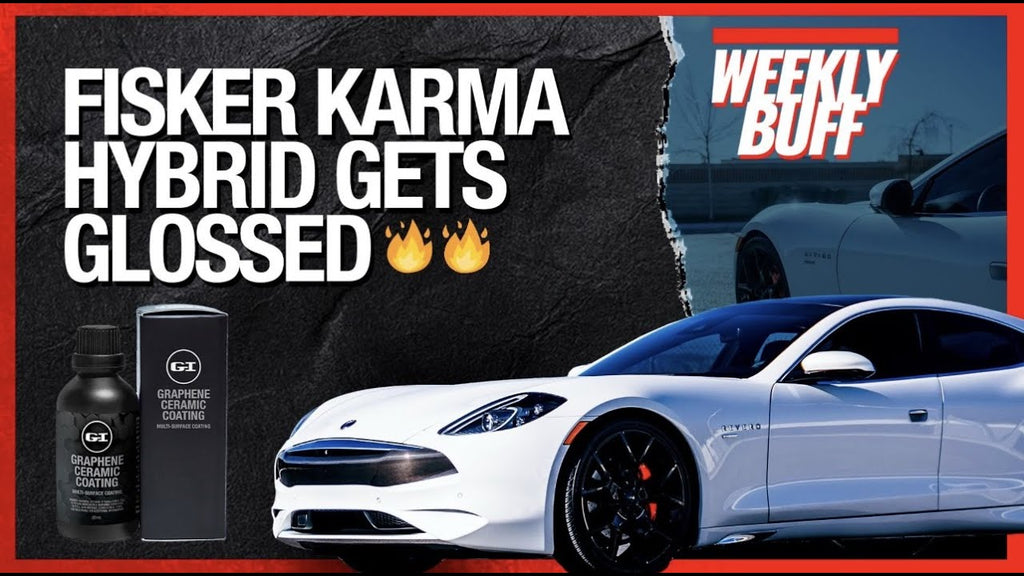This advertisement, enclosed within a horizontal rectangular frame featuring a red border, showcases the Fisker Karma Hybrid in a visually striking and detailed manner. The focus is on a sleek, white streamlined sports car occupying the bottom half and right two-thirds of the frame. In the upper left-hand corner, bold white uppercase text proclaims “Fisker Karma Hybrid Gets Glossed,” accented with two fire emojis. Additionally, the phrase “Weekly Buff” appears prominently, enhancing the car’s pristine appeal. 

On the lower left side, the advertisement highlights the product: a black bottle of Graphene Ceramic Coating alongside its matching black box, both adorned with white text reading "Graphene Ceramic Coating" and featuring the GI circular logo. Together, these visual elements emphasize the car's glossy finish and the efficacy of the advanced ceramic coating product, crafting an enticing call to automotive enthusiasts and perfectionists alike.